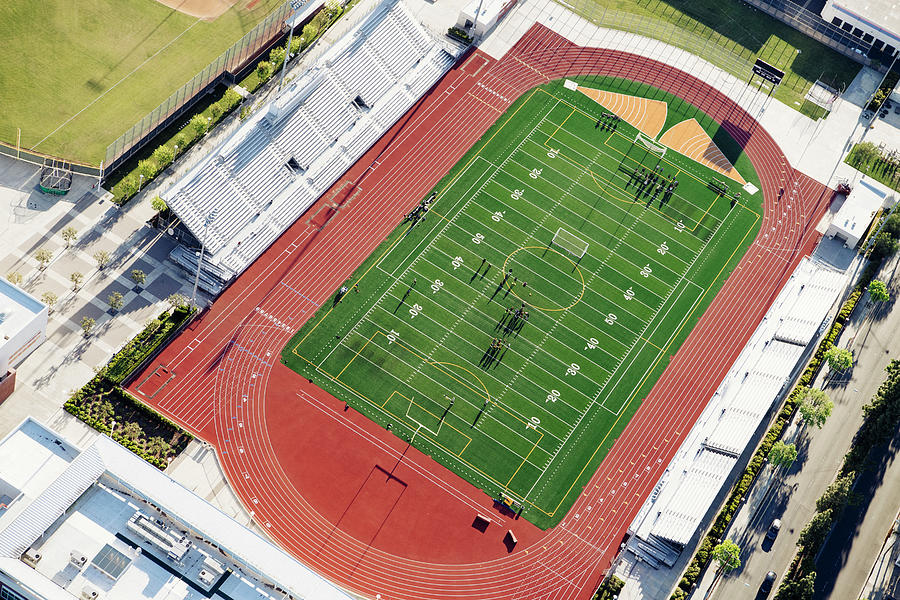The photograph showcases an aerial view of what appears to be a high school or college multi-purpose athletic stadium. Dominating the center is a green football field marked with white lines for American football and yellow lines for soccer. Surrounding the field is a reddish-brown, circular running track, which also includes a straight sprint track. The stadium features white or silver bleacher seats on both sides, all empty, indicating no ongoing event. Scattered groups of people are on the field, with clusters near the 20-30 yard line and around the end zones, possibly indicating a practice session. To the left of the track is a grassy area, and beyond the stadium, at the top of the image, are some buildings, while a street runs along the right side. There appears to be a potential baseball field to the left, identifiable by sandy areas. A walkway lined with little trees leads out of the track area, connecting to a white building.